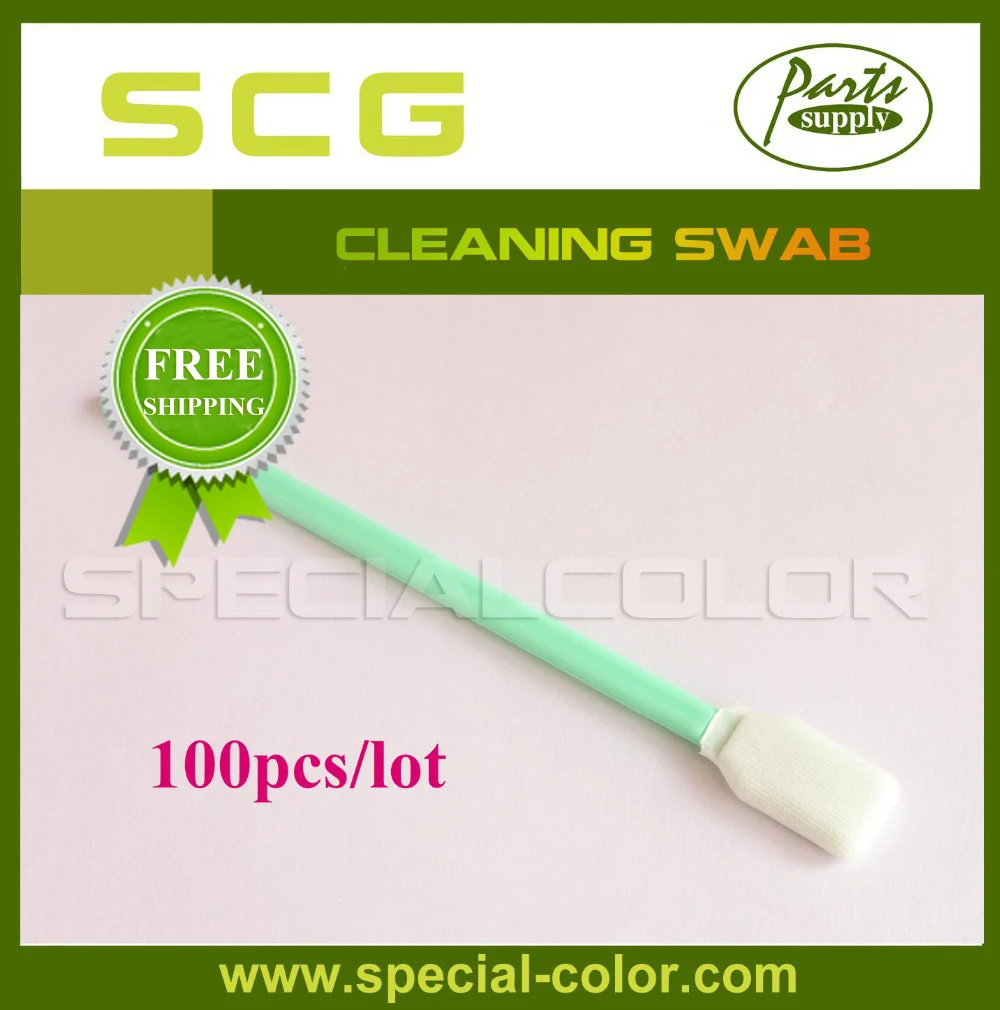This image is an advertisement for a cleaning swab. The design is bordered in dark green, with the bottom border in a lighter yellow-green, displaying the website www.special-color.com. At the top, the text "SCG" is written in olive green, followed by "Parts Supply". An oval logo appears to the right, further indicating that the company specializes in parts. A horizontal green bar spans the image with gradients flowing into orange and red, highlighting the text "Cleaning Swab". On the left, there's a graphical element resembling an award ribbon in green and white, with the text "Free Shipping". The featured cleaning swab, thin and light green with a white tip, is shown at a diagonal. Superimposed over the swab in white text is "Special Color". Below the swab, the red text reads "100PCS4-LOT". The main colors of the advertisement are shades of green, accented with white, orange, and red.